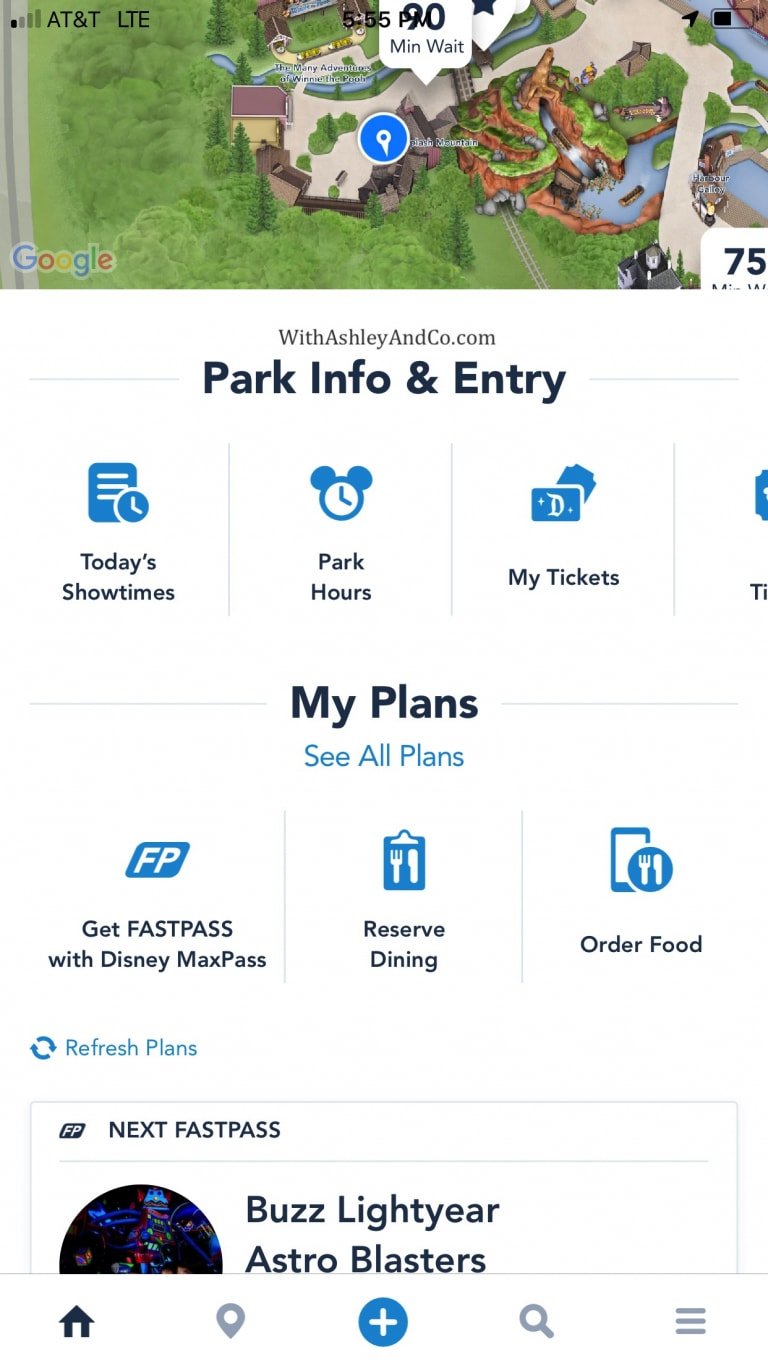The image captures a smartphone displaying a detailed webpage. The phone has a partially charged battery and operates on AT&T’s LTE network, but is not currently connected to Wi-Fi. The header of the webpage features an aerial illustration depicting a residential cul-de-sac surrounded by water bodies, trails, trees, grassy areas, and forests. A blue circular marker with a white pin designates a specific location on this map, which is confirmed to be from Google Maps by the Google watermark in the lower left-hand corner. The lower right corner shows "75 something" and provides access to park information under "Ashleyandcompany.com."

The central section of the page lists various features starting with "Today's Showtimes," "Park Hours," and "My Tickets," each accompanied by blue icons. "My Plans" includes links for "See All Plans," "Get Fast Pass with Disney," "Max Fast Pass," "Reserve Dining," and "Order Food," all featuring corresponding blue icons. The section concludes with options to "Refresh Plans" and information on the "Next Fast Pass," which is for "Buzz Lightyear Astro Blasters." Below, standard navigation icons are displayed at the bottom of the screen.